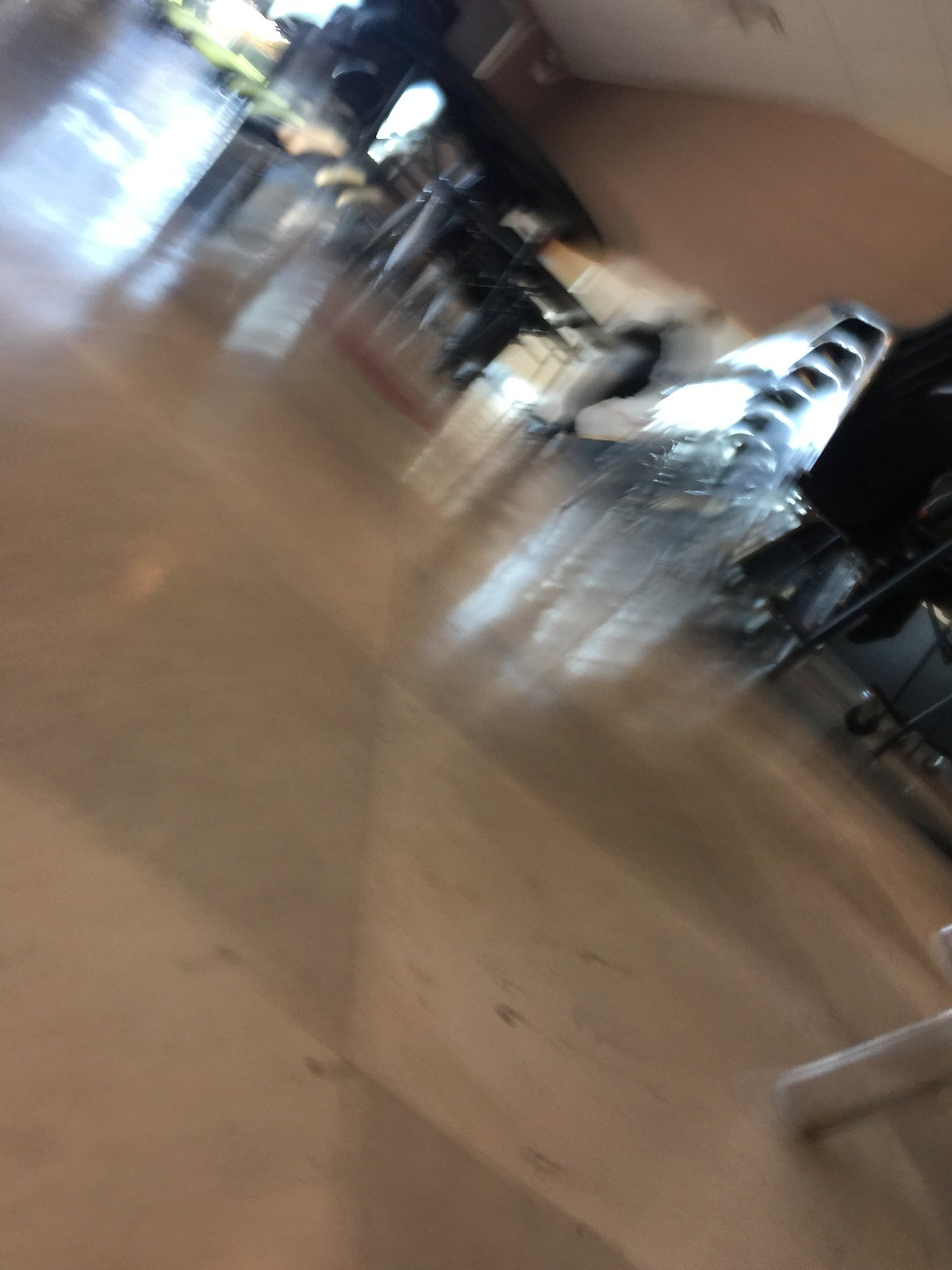This incredibly blurry photo appears to have been taken indoors on a floor composed of alternating light brown and dark brown square tiles. The image is tilted at an angle, running from the upper left to the lower right. In the upper left corner, there's a window with sunlight reflecting off the floor. To the right of the window stands a round black table supported by a gray platform. Nearby, on the right side of the photo, part of the medium brown-colored wall is visible, along with some kind of gray object, potentially another window, reflecting light from the floor. In the lower right corner, a metallic object, possibly the leg of a chair, is discernible. The background features indistinct areas of bright silver and black, which might be stacked chairs or miscellaneous items, suggesting the setting could be a cafeteria.